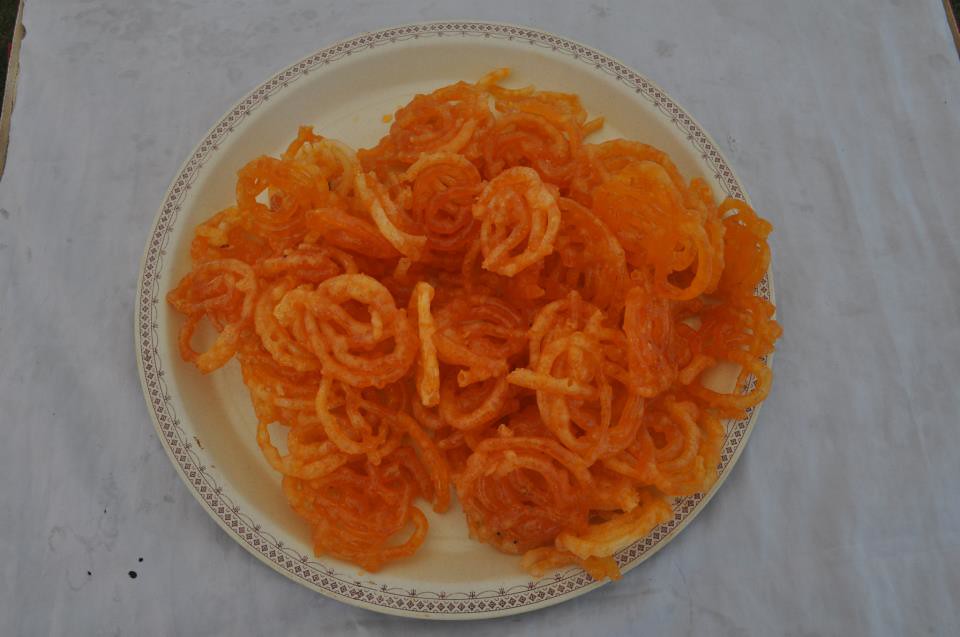This photo depicts a white or cream-colored plate featuring a light red or brown geometric border, set upon a coarse, off-white tablecloth. The tablecloth covers most of the table, with only a hint of wood visible at the very edges. On the plate, there is a serving of orange, curly, spiral-shaped items, which could be curly fries, fried vegetables, or cheese crisps, given their fried or baked appearance with varying hues of orange. The texture suggests they might be crispy, while the moist sheen indicates possible dampness.